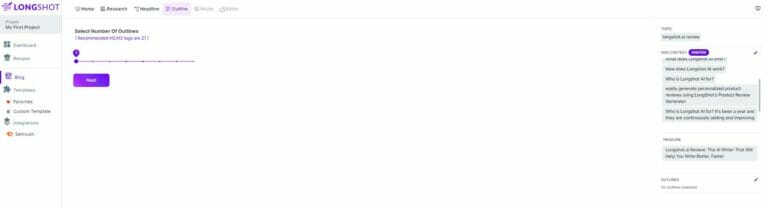The image is a screenshot of a website's interface. At the top left corner, there's a purple text that reads "Long Shot". Adjacent to this are six clickable areas, numbered 1 through 6. Along the left side of the page, there's a vertical column filled with various icons, each accompanied by text labels, although the small size of the image makes the text difficult to read. In the middle of the page, there's a prominent purple dot centrally placed, surrounded by seven interactive areas that allow the dot to be moved towards the right. Below this, a purple button with white text is visible, but the specific wording is unreadable. On the far right side, the page appears to contain text input areas, with one noticeable purple button in the second section, followed by additional text boxes and spaces further down the page. The overall design features a dominant purple color scheme and a structured layout for navigation.